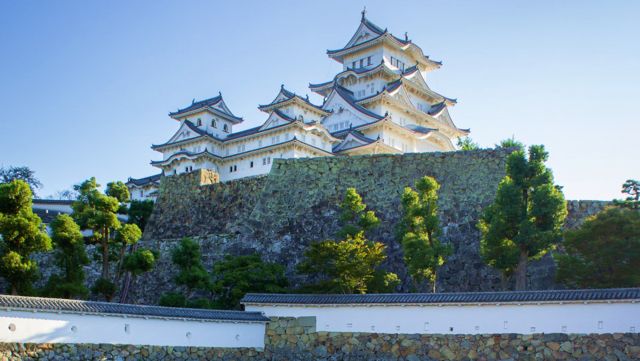The image captures a striking example of traditional Chinese architecture, featuring a massive, intricately designed structure enclosed by an imposing stone wall. The wide-angle photo highlights the building's multi-tiered, pointed roofs and abundant windows, which are bathed in sunlight from the right side of the frame. This sunlight casts a warm glow over the lush trees lining the base of the fortress-like stone wall, which appears robust with a thickness of at least six feet at the top, potentially doubling at the bottom. The sky overhead transitions from a deeper blue in the left-hand corner to a lighter hue, providing a picturesque backdrop. The stone wall, interspersed with patches of green tones, supports a variety of trees and bushes. Nearer to the photographer, a lower stone fence with wooden beams adds to the scene's intricate details. The structure's architecture, distinguished by its turned-up roof corners and multiple roof levels—six on the tallest section and three or four on the shorter side—suggests it may be a significant building, possibly even a hotel, situated in China.